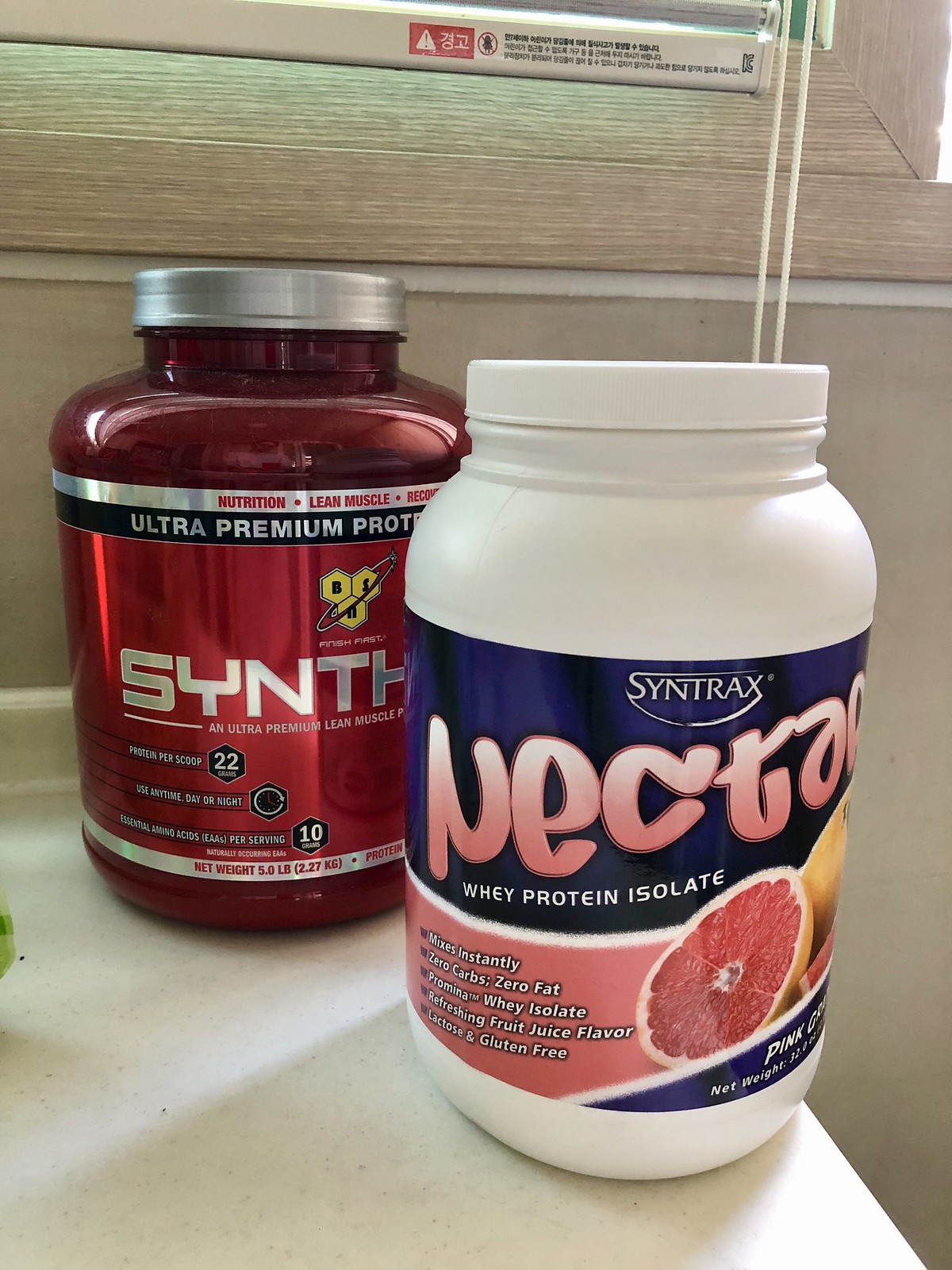This detailed photograph depicts two large canisters of food supplements placed on a white countertop within an Asian household, as indicated by the Chinese writing on the bottom of the blinds in the background. The setup includes a wooden windowsill and blinds hanging down with a white string to open and close them. 

The first canister, prominently white with a label in purple and pink, is from the Syntrax brand. It features the word "Nectar" and is labeled as a Whey Protein Isolate with a pink grapefruit flavor. This tub boasts various health claims, including being lactose and gluten-free, having zero carbs and zero fat, mixing instantly, and promoting lean muscle recovery with Promina TM whey isolate.

The second canister is strikingly red with a silver lid, originating from the Synthasix brand. Its label highlights it as an Ultra Premium Protein supplement designed for lean muscle recovery, offering 22 grams of protein per scoop and containing 10 essential amino acids per serving. The product's net weight is specified as 5.0 pounds, catering to those focused on muscle nourishment and overall fitness.